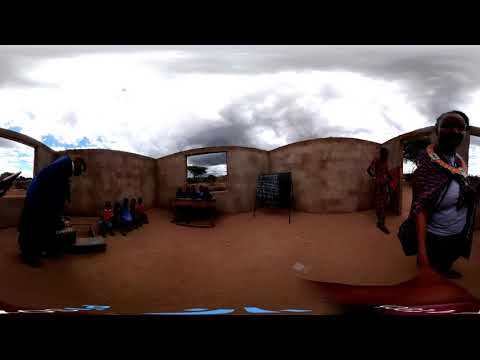In this image taken outdoors, the scene is set within a partially constructed environment featuring only walls that curve and connect to each other, with no ceiling or roof. The walls are white and tan, hinting at an arid, possibly desert location. Openings in the walls serve as windows and doorways, but there are no actual windows or doors. The floor appears to be dirt. The sky above is detailed with fluffy white and gray clouds, and there's a brighter area in the left corner suggesting the presence of the Sun, which is not directly visible.

There are multiple people in the image. On the left, a man wearing a blue suit or gown is bending down, seemingly interacting with a brown and black object on the ground. Nearby, five children are seated on a bench, dressed in various colors ranging from red to black to blue. Additionally, there’s a wooden table beside them, holding unidentified items. Beyond them, a chalkboard stands, black with white chalk writing.

To the right of the children, a woman in a blue t-shirt and a cape-like purplish shawl is reaching down toward something unseen. She sports a distinctive orange ring around her neck, and her face appears blurred or blacked out, making her features difficult to discern. There is another person dressed in a red and white plaid outfit standing nearby, whose gender is indistinct. In the background, visible through the window openings, are expansive views of the sky and a distant tree, reinforcing the outdoor setting.